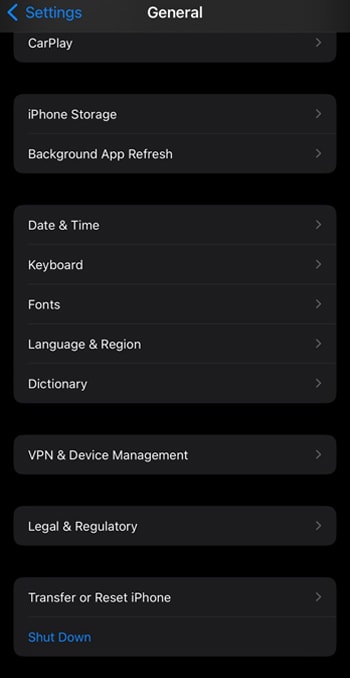This image is a screenshot of a phone's settings menu. At the top left corner, there is a back arrow followed by the word "Settings" in blue. The general theme of the background is various shades of black and gray. Centered at the top of the screen, the word "General" is displayed in white text. Below "General" is a list of options, each accompanied by a right-facing arrow to indicate further details can be accessed:

1. CarPlay
2. iPhone Storage
3. Background App Refresh
4. Date & Time
5. Keyboard
6. Fonts
7. Language & Region
8. Dictionary
9. VPN & Device Management
10. Legal & Regulatory
11. Transfer or Reset iPhone

These options are displayed in white text against a lighter black segment of the background. At the very bottom of the screen, the "Shut Down" option is highlighted in blue. The rest of the menu items remain in white text. There are no visible indicators of the phone's current date, time, or battery status, as those elements are out of the screenshot's frame. Overall, the image features mostly monochrome elements, with the only accents being the blue color for "Settings" and "Shut Down."